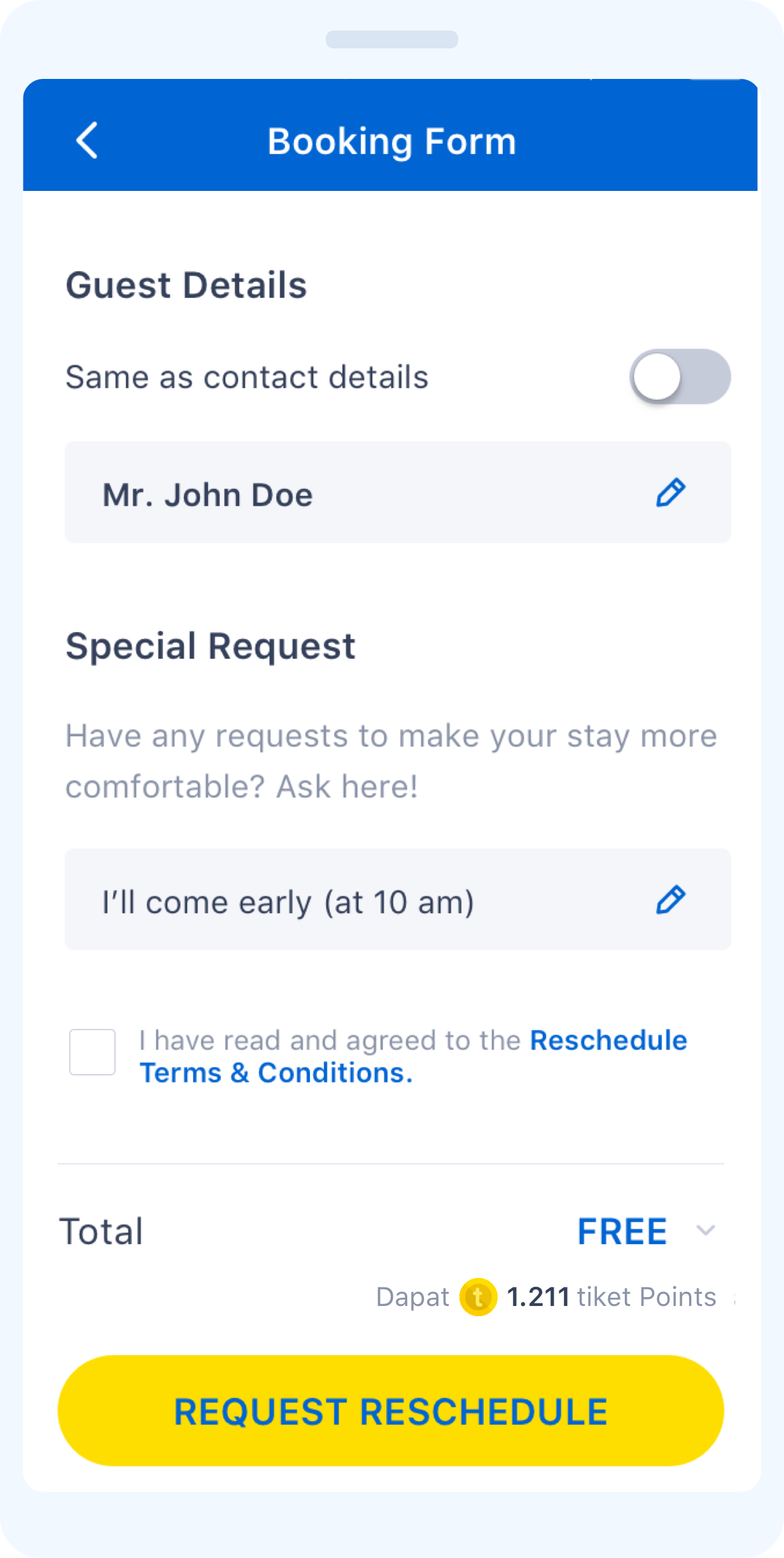The image is a screen capture from a cell phone, displayed in a rectangular format with the larger side aligned vertically. The top of the screen features a blue banner displaying the text "Booking Form" in white letters centered in the middle. To the left of this text, there's an arrow icon pointing to the left.

Below the blue banner, the background transitions to white with black text that reads "Guest Details." Underneath, in gray letters, it states "Same as Contact Details," next to an oval switch which is currently turned off. 

Following this, there are details about the guest, starting with the name "John Doe" formatted as "Mr. John Doe," accompanied by a blue pencil icon to the right, indicating an option for editing. 

Further down, in black letters, the text "Special Request" is displayed, with a gray instructional note just below it that says, "Have Any Requests to Make Your First Day More Comfortable, Ask Here!" Below this, a lightly gray-filled oval input box is available, containing the text "All Come Early (10 a.m.)" in black letters. There is another blue pencil icon on the right of this input box for editing purposes.

Continuing downward, an unchecked checkbox appears next to the text "I Have Read and Agreed to the Reschedule Terms and Conditions." 

A light gray bar thereafter serves as a separator, under which the word "Total" is displayed in black letters. Adjacent to this, the word "Free" appears in uppercase blue letters.

At the bottom of the screen capture, there is a solid yellow oval button with blue text in capital letters that reads "REQUEST RESCHEDULE."